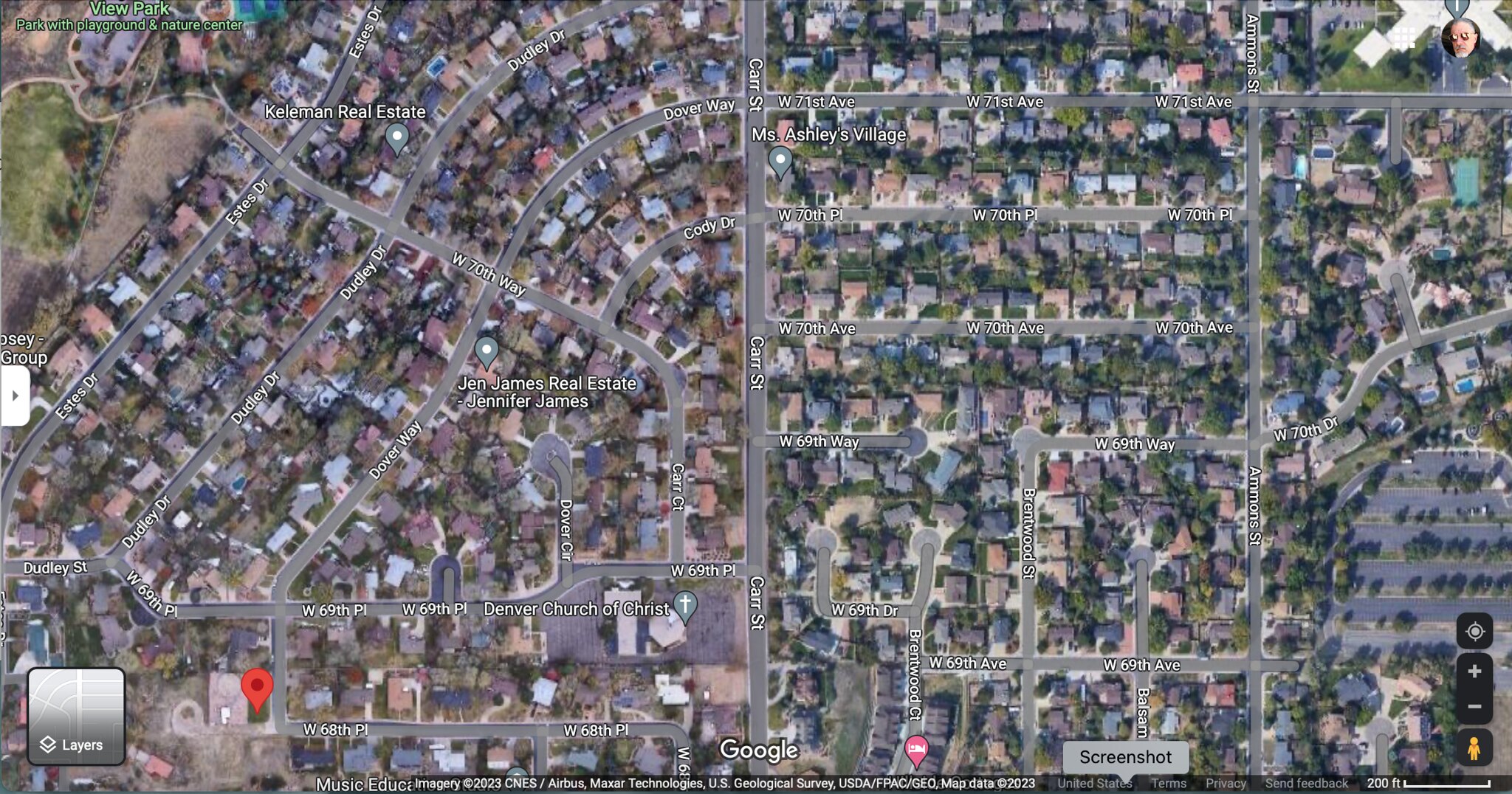This is an aerial view image obtained from Google Maps, showcasing a diverse landscape intersected by a prominent road running vertically. The screenshot, as indicated by the Google Maps watermark at the bottom, highlights distinct differences in the land on either side of the road. To the right, the terrain takes on a brownish hue, suggestive of barren land or minimal vegetation, while the left side is lush and green, likely due to dense tree coverage.

Prominent black roads crisscross the landscape, with a notable intersection where the main vertical road divides into differently appearing streets. In the upper left-hand corner, "View Park" is labeled, suggesting a point of interest for navigation. Various icons and labels mark notable places, including a red balloon marker indicating a chosen destination.

In the upper right-hand corner of the image, there's a small picture of a person with glasses, possibly the user account on Google. The lower left corner shows the word "Layers," indicative of the map's layer options. Additionally, the image identifies a nearby park, a real estate office, and a church, among other labeled points of interest, offering a clear, comprehensive overview of the area.